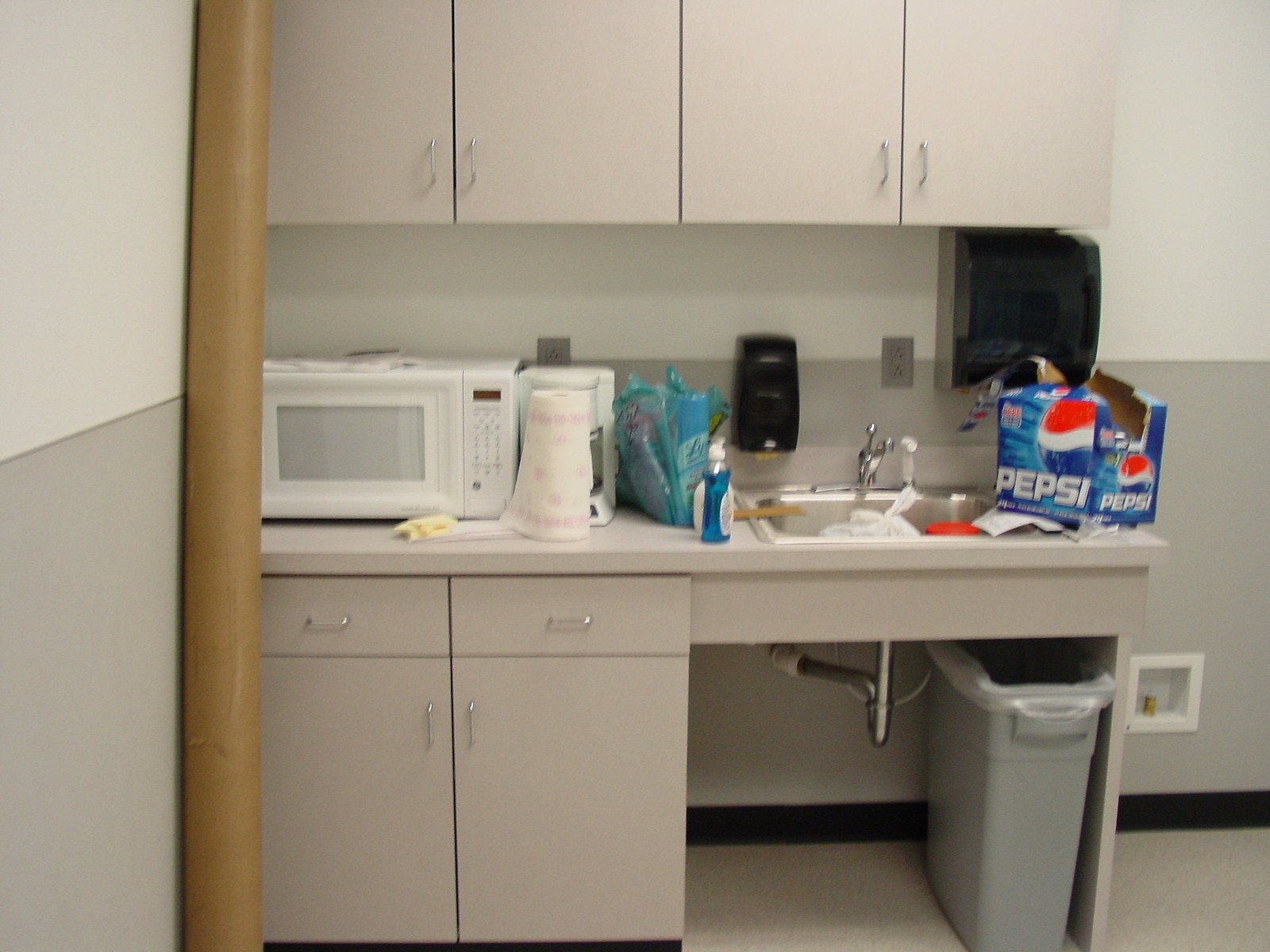The photograph showcases a cluttered work area featuring a mixture of cabinetry and various items strewn across the countertop. Overhead, there are four cabinet doors with sleek silver handles. Below, two cabinets sit to the left, and to the right an open space accommodates the stainless steel sink. On the left side beneath the countertop, two large rectangular cabinets are positioned beneath a pair of drawers.

The counter itself is strewn with various items. On the far right, an empty Pepsi box sits next to the stainless steel sink, which features a single-knob faucet. Mounted on the wall between the sink and the upper cabinets is a black paper towel dispenser, and to the left of the sink, a black soap dispenser is affixed to the wall. To the immediate left of the sink is another hand soap pump and a roll of paper towels.

Behind these items, a small, white single-serve coffee pot is visible. Further to the left, a white microwave rests on the counter with several towels laid in front of it. The scene is one of active use, with a variety of functional and everyday items contributing to the busy atmosphere of the workspace.